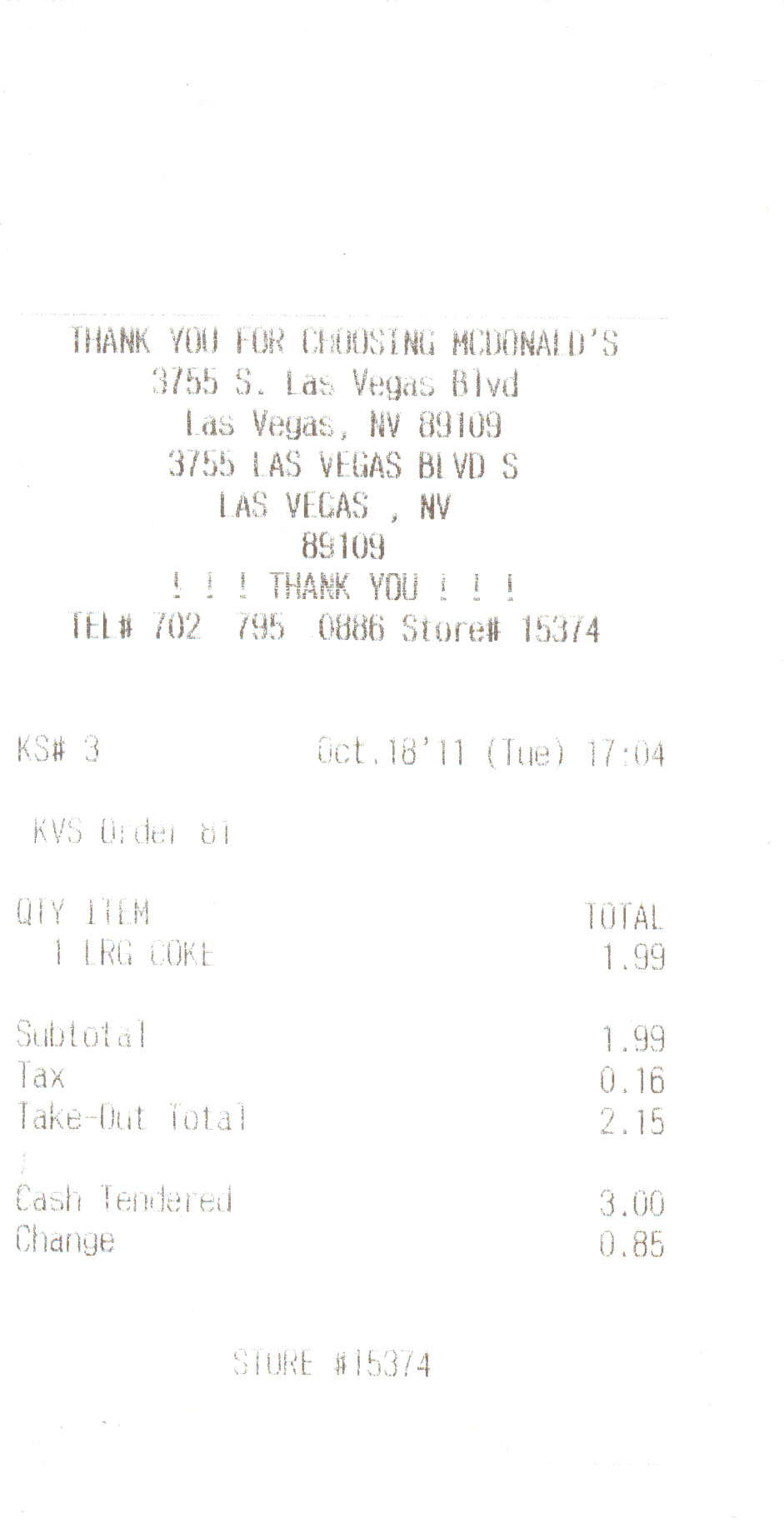This image depicts a slightly faded receipt printed on white paper from a McDonald's. The text is in black ink, suggesting the printer was low on ink. At the top, the receipt reads, "Thank you for choosing McDonald's," followed by the store's address, phone number (702-795-0886), and store number (15374). It is dated Tuesday, October 18, 2011, at 17:04. The purchase detailed on the receipt is one large Coke, costing $2.15 after taxes. The customer paid with $3.00 and received 85 cents in change.